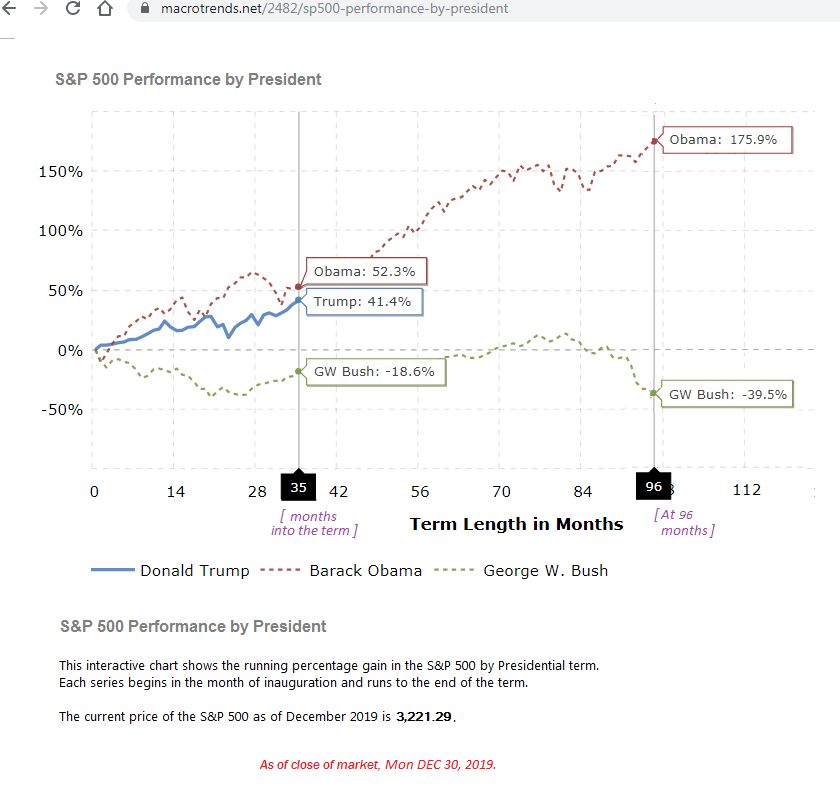The image is a detailed computer-generated screenshot depicting a graph titled "S&P 500 Performance by President" against a white background. The Y-axis on the left displays percentages marked at intervals of -50%, 0%, 50%, 100%, and 150%, while the X-axis shows the time in months, marked at 0, 14, 28, 35, 42, 56, 70, 84, 96, and 112. The graph features three distinct lines representing the performance of the S&P 500 under Presidents Obama, Trump, and George W. Bush, with different colors for each.

- Obama: Represented by a red dotted line, showing a significant increase, peaking at 52.3% at 35 months and reaching 179.9% at 96 months.
- Trump: Depicted by a solid blue line, showing a performance gain of 41.4%.
- George W. Bush: Shown with a green dotted line, indicating a decline, marked at -18.6% initially and dropping further to -39.5%.

Additional text at the bottom of the chart states, "This interactive chart shows the running percentage gain in the S&P 500 by presidential term," along with the closing market date of Monday, December 30, 2019, and the S&P 500 price of 3,221.29. Text colors vary, with black and gray for the main content and red for the closing date.